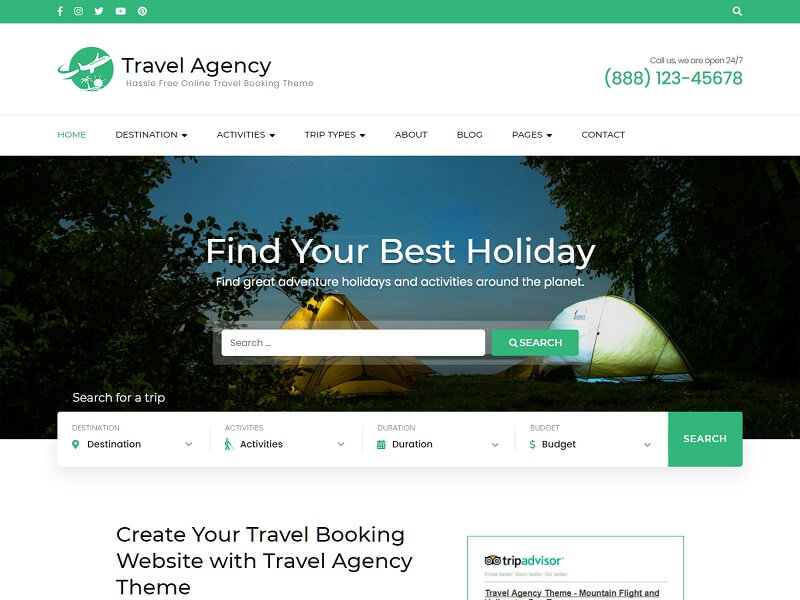This is a screenshot of a website designed as a sample travel agency platform. At the top of the page is a leaf-green banner adorned with white social media icons for Facebook, Instagram, Twitter, YouTube, and Pinterest, followed by a white magnifying glass icon on the right for search functionality.

Below the banner, there is a prominent white rectangle featuring a green circular icon with a white airplane flying over a palm tree. Next to this icon, in bold black font, is the text "Travel Agency." Directly beneath that, in gray font, is the tagline "Hassle-Free Online Travel Booking Theme." To the right of this section, a message reads, "Call us, we're open 24/7," followed by a placeholder phone number, "888-123-45678," indicating that this example is not for a real company but rather a prototype.

Further below, the navigation menu includes dropdown options labeled Home, Destination, Activities, Trip Types, About, Blog, Pages, and Contact, offering a comprehensive structure for how the website could be organized. This mockup effectively demonstrates how to design and build a user-friendly travel booking website.